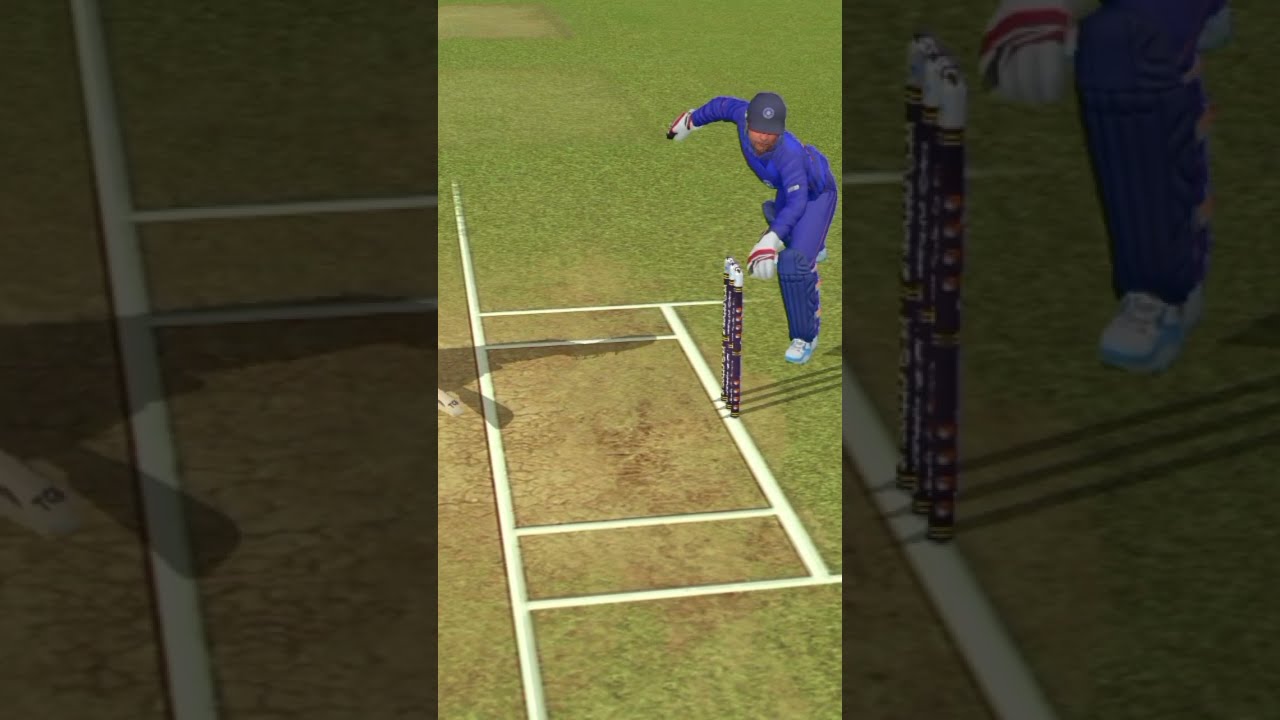The image depicts a man in the middle of a cricket field, dressed in a blue athletic uniform with long sleeves and long pants, accompanied by white gloves and a gray hat or helmet. To his side are three vertical stakes, known as wickets, indicative of the game of cricket. The field displays white lines demarcating the play area on a mix of green grass and a small brown patch, which confirms the setting as a cricket pitch. The central third of the image is in sharp focus on the man and the wickets, while the left third features an out-of-focus, grayed-out spectator. The main colors of the image are green, white, and blue. The man's right arm is positioned behind him, suggesting he might be about to bowl or field, enhancing the dynamic essence of the scene.